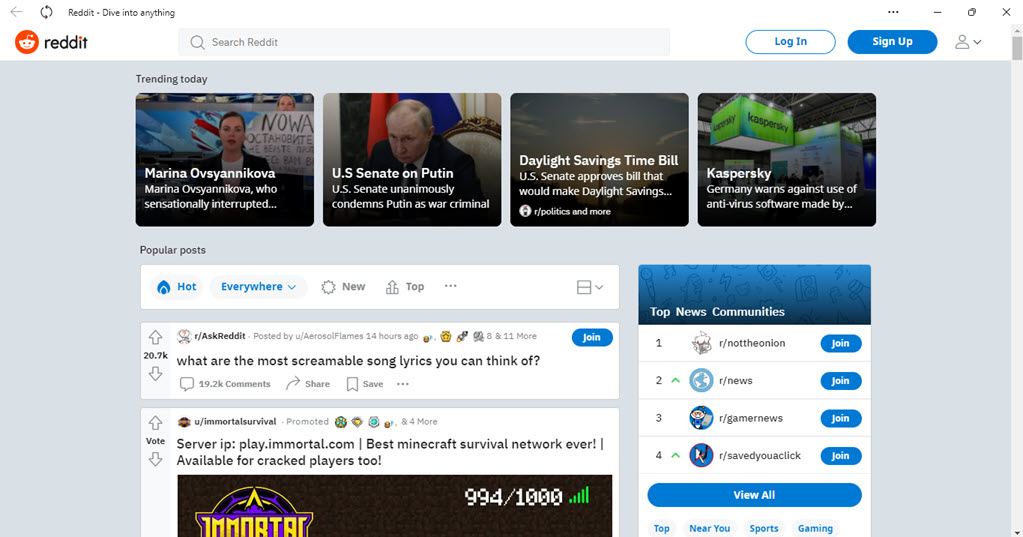The image displays a Reddit webpage. At the top left corner, the familiar Reddit logo is visible. To its right, a search bar is prominently displayed with the placeholder text "Search Reddit." Continuing to the right, there are buttons labeled "Log In" and "Sign Up."

Below this header section, trending articles are highlighted. The first article features a picture of a young woman named Mariana Ossanikova, suggesting the article is centered around her. Next to it is an image of Vladimir Putin, accompanied by a headline that reads, "U.S. Senate: U.S. Senate unanimously condemns Putin as a war criminal." Following this, a photograph of a sky precedes a headline about a daylight savings time bill, indicating that the U.S. Senate has approved a bill related to daylight savings time. The last article in this series shows a headline about Kaspersky, noting that Germany warns against using the anti-virus software.

Further down the page, various Reddit posts are visible. One from the AskReddit community poses the question, "What are the most screamable song lyrics you can think of?" Another post, marked as an ad, promotes "The Best Minecraft Survival Network Ever."

This detailed view captures the typical layout and range of content presented on Reddit's homepage.